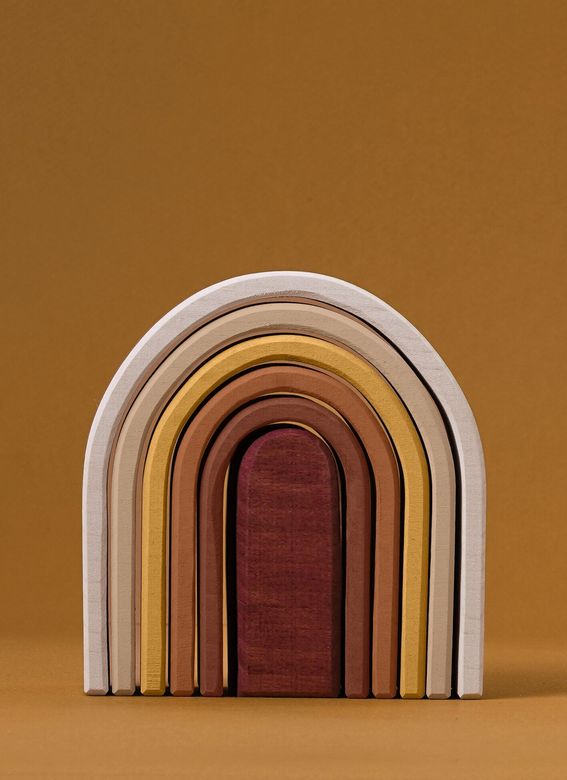This photograph showcases a modern interpretation of a rainbow design, where thick, U-shaped arches made from either clay or wood are meticulously arranged. The rainbow consists of five distinct, progressively larger bands surrounding a solid, dark cherry wood piece at the center. The colors of the bands, from outermost to innermost, are white, tan, yellow, brown, and dark brown, culminating in the dark centerpiece that matches the innermost arch. The entire structure is set against a modern light brown background, casting a shadow to the right. The cohesive play of earthy tones and robust materials provides a contemporary yet natural aesthetic.